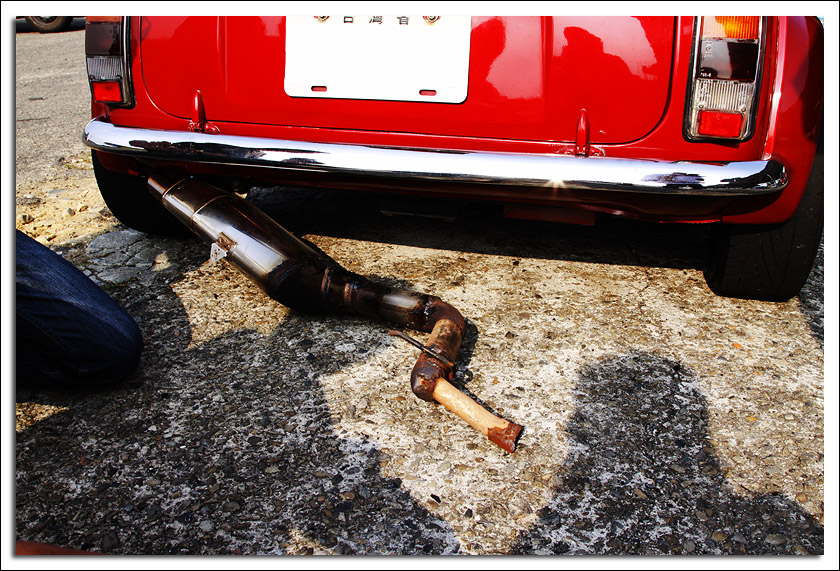This image captures the back end of a shiny red car, stopping right at the taillights and showcasing a significant problem: the muffler is falling off, hanging down and touching the ground. The car, detailed with a silver metallic bumper and characterized by brown and tan rust creeping onto the muffler, sits on a rocky pavement. To the left, part of a person's leg is visible, possibly indicating someone kneeling next to the vehicle. The license plate area is empty and white. The scene includes slight shadows, enhancing the metallic sheen of the bumper and the neglected state of the exhaust system.